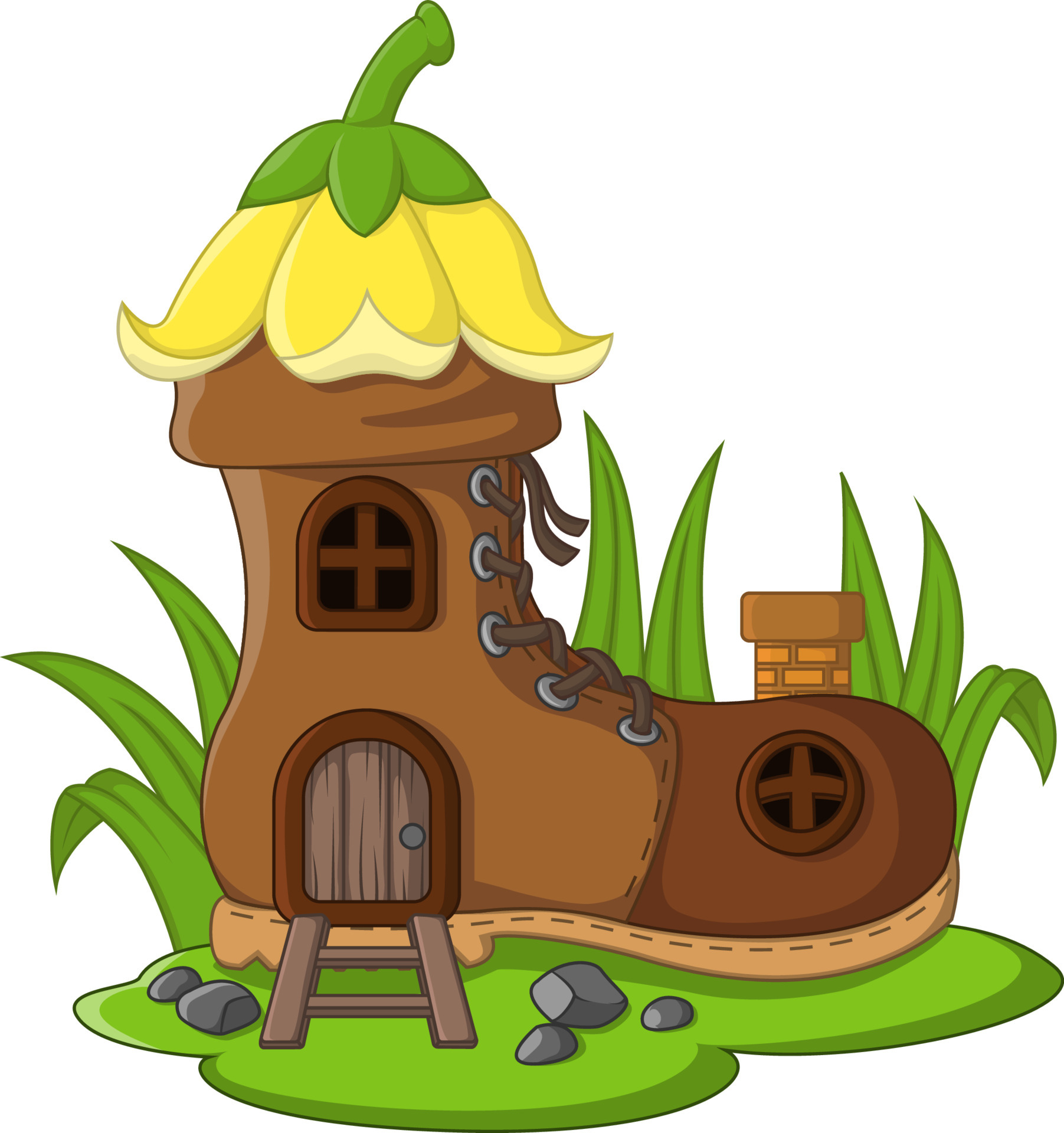This is a detailed, hand-drawn cartoon illustration of a large, old boot that has been transformed into a whimsical house. The boot, sitting in a patch of green grass with taller grass surrounding it, faces to the right with its heel on the left. The predominantly light brown boot features a darker brown toe and laces, along with a lighter brown heel. A wooden door, trimmed in dark brown and located where the heel is, serves as the entrance to this fantastical home. The door is arched, has a doorknob, and is accessed by a small set of wooden stairs. Above the door, an arched window with a dark brown frame and a cross pattern complements a similar, round window situated near the toe of the boot. Topping off this imaginative structure is an upside-down, yellow flower with a green stem, acting as the roof. Additionally, a lighter brown chimney with tan bricks emerges from the upper front of the shoe, adding to its house-like charm. The background of the image is a plain white, emphasizing the detailed and colorful elements of the boot house.